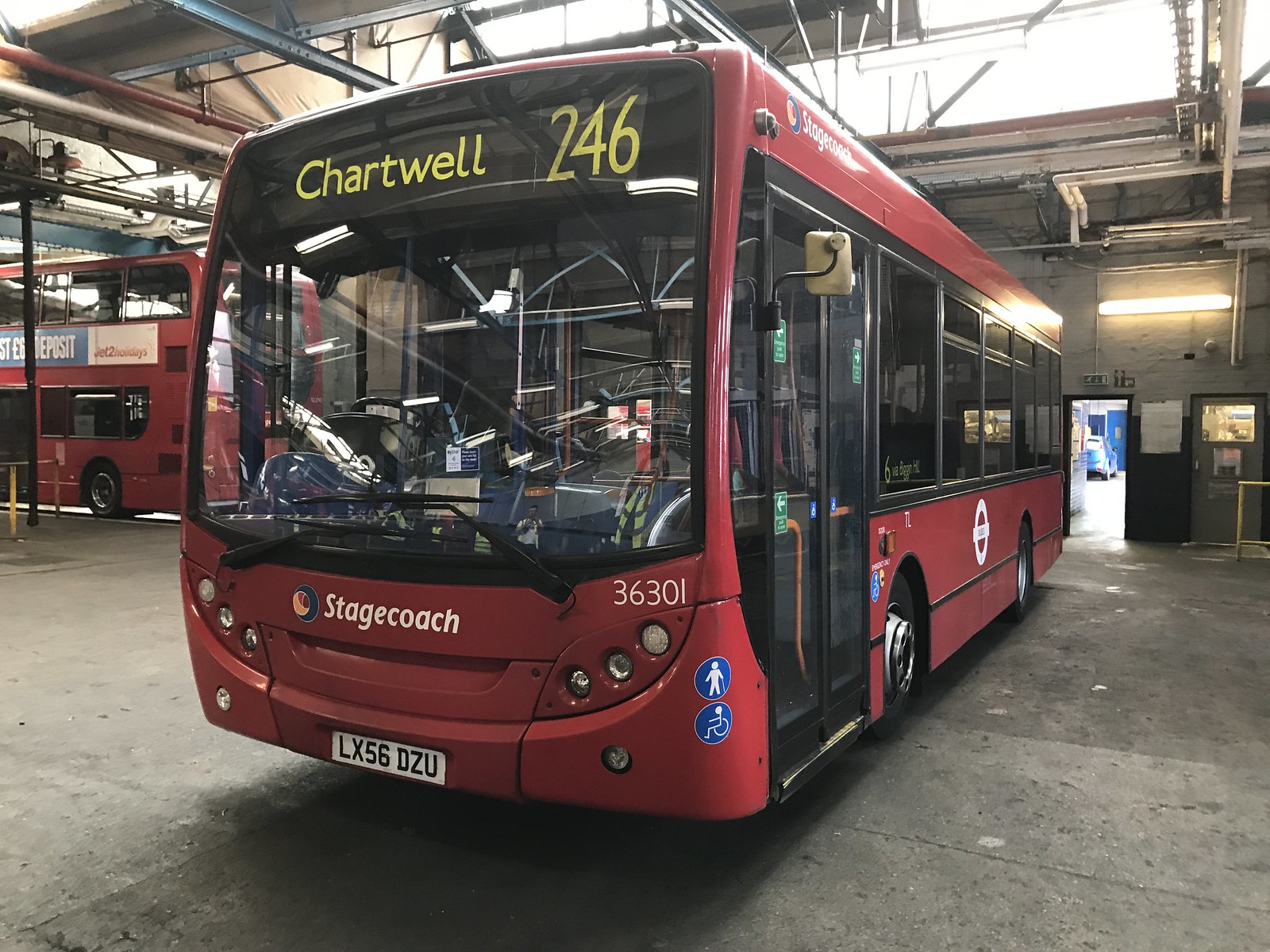The image depicts the interior of a bus garage housing several vehicles, including a prominently featured single-decker Stagecoach shuttle bus in the foreground. This shuttle bus, identified by its route number "Chartwell 246" displayed on a digital sign at the front, is visually striking with its bright red exterior and upper body predominantly composed of windows. The bus bears the number 36301 and displays the license plate LX56DZU. Notably, it is handicap accessible, marked by visible stickers on the front and side, and features see-through doors adorned with green signs featuring white text.

In the background, another red bus, which appears to be a double-decker, carries a banner advertising “Jet 2 Holidays” and mentioning a £6 deposit. Additionally, a blue car is visible further back in the garage area. The scene is set within a spacious interior where the buses are presumably maintained and prepared for their routes.